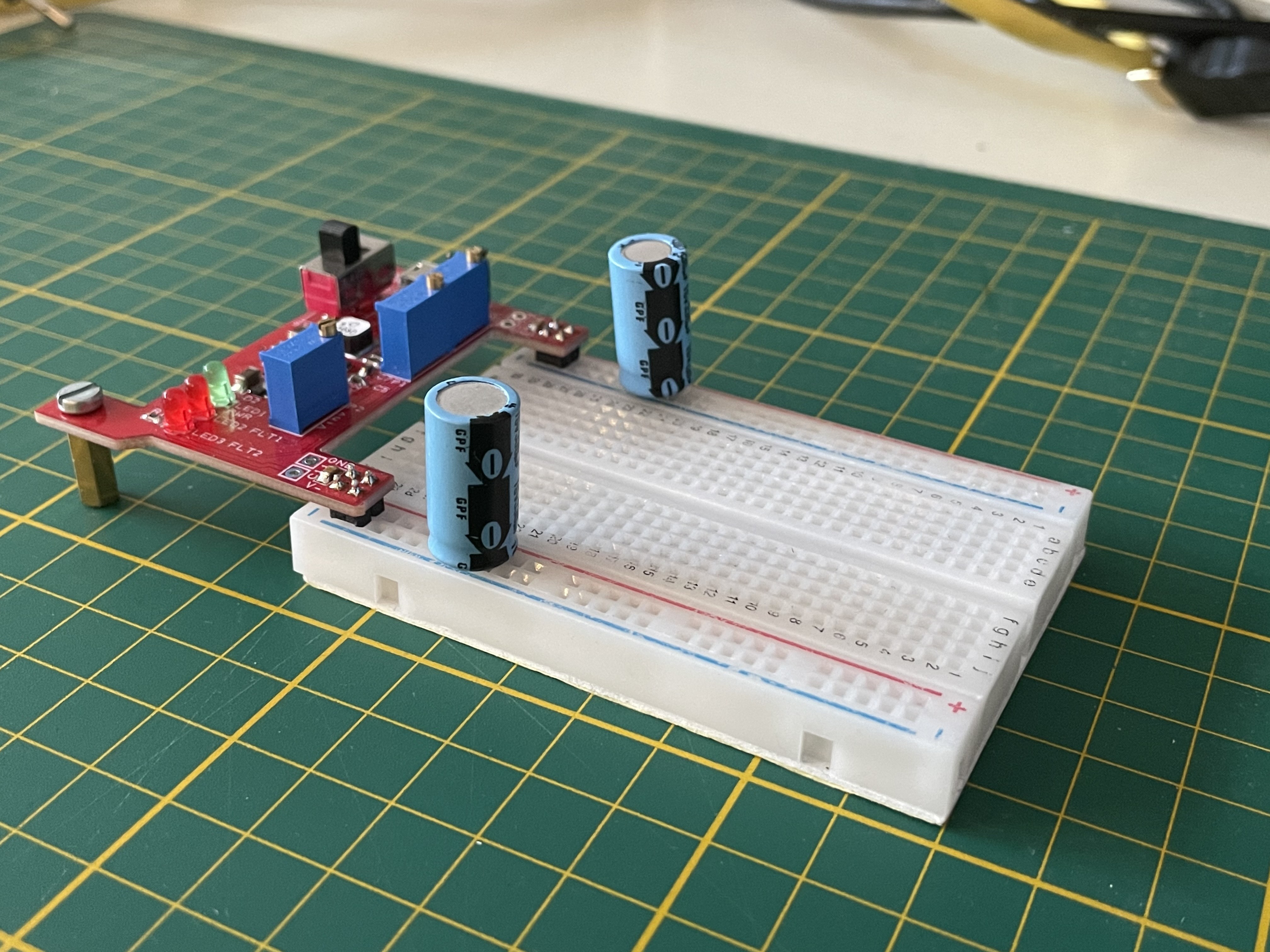This image captures a detailed setup of a red circuit board, which includes blue and black components and is equipped with two round batteries on either side of a white, perforated section into which the board is plugged. The circuit board, potentially a power supply circuit, also features two small red lights and one green light. It is situated on a green cutting mat characterized by evenly spaced yellow squares formed by intersecting horizontal and vertical lines. The scene occupies the left side of the mat, leaving a notable empty space on the right. The backdrop includes parts of a workbench or workshop table, with a blurred background featuring an indistinct beige object positioned in the upper right corner. The overall setting suggests a meticulous and organized workspace.